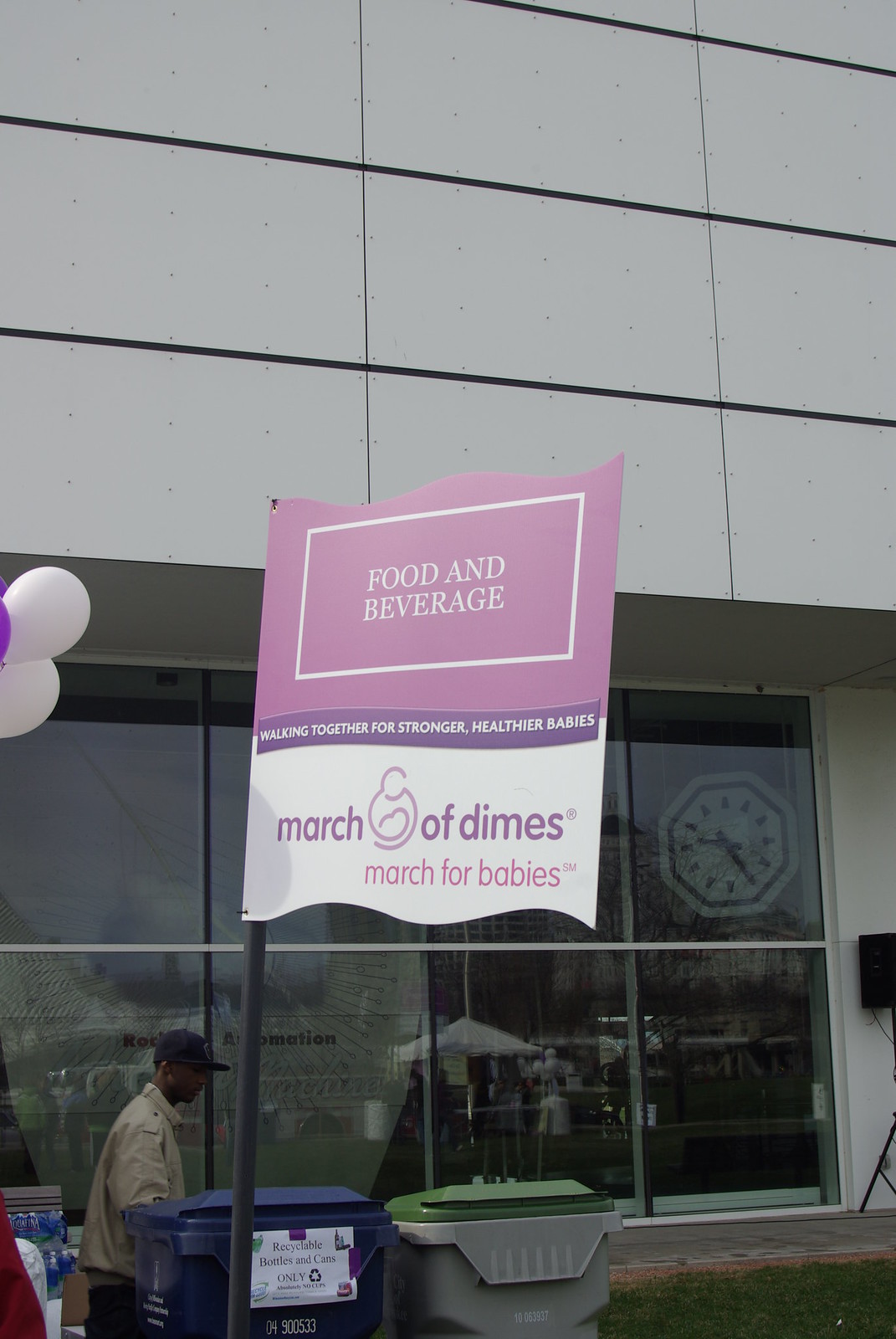The image depicts the front of a building with a prominently displayed sign in the foreground. The sign, attached to a gray metal pole via black zip ties at the bottom left and top left corners, is divided into two sections. The top half of the sign is purple, featuring a white-bordered rectangle with "Food and Beverage" written in white font against a purple background. The bottom half is white with "March of Dimes March for Babies" written in purple. A purple banner with the white text "Walking Together for Stronger, Healthier Babies" separates the two sections.

In front of the signpost, there are two trash cans; the left one is blue, and the right one is gray with a green lid. Behind the sign, a black man wearing a black hat and a beige jacket stands near the two bins, which might be for donations. The building in the background features a glass front, through which an interior clock with no numbers, only dots, is visible.